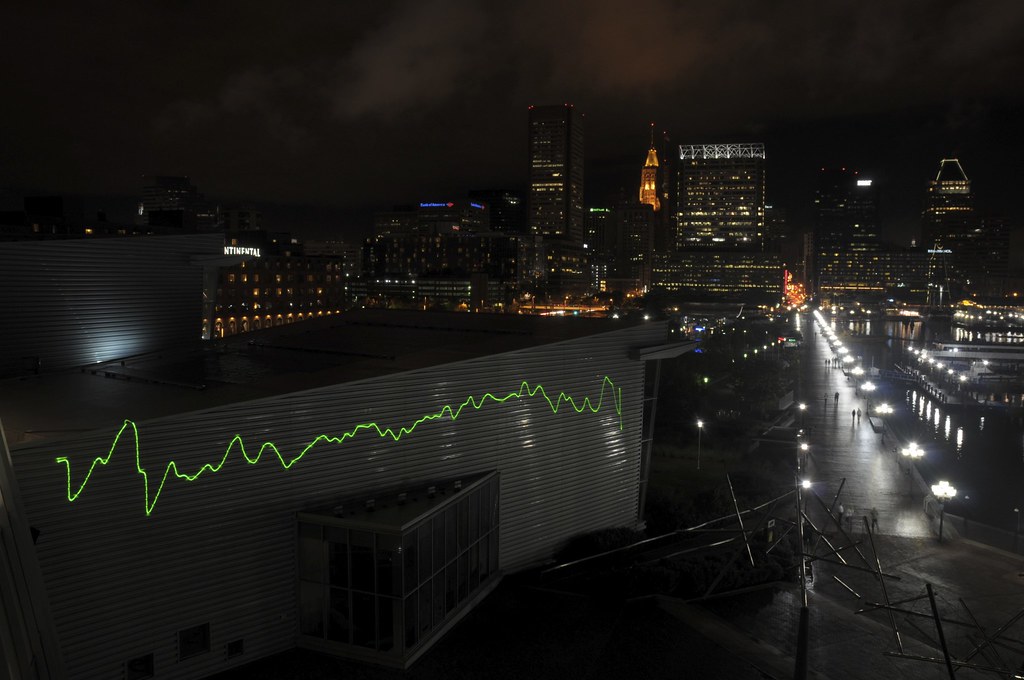This is a photorealistic nighttime cityscape featuring a dark, cloud-streaked sky. In the background, the outlines of several skyscrapers and high-rise buildings are illuminated by lit-up windows. On the right side of the image, a street runs along a boardwalk with barely discernible figures walking beneath bright streetlights. The figures appear to be on a bridge extending over a reflective water source, possibly a river or canal. On the left side, a large corrugated metal building, reminiscent of a warehouse, is prominently marked by a jagged bright green line that evokes the appearance of a heartbeat monitor's reading. This mysterious green line adds an enigmatic element to the scene. The overall color palette of the image is quite dark, with light sources concentrated on the buildings and streetlights, creating a stark contrast against the night sky.